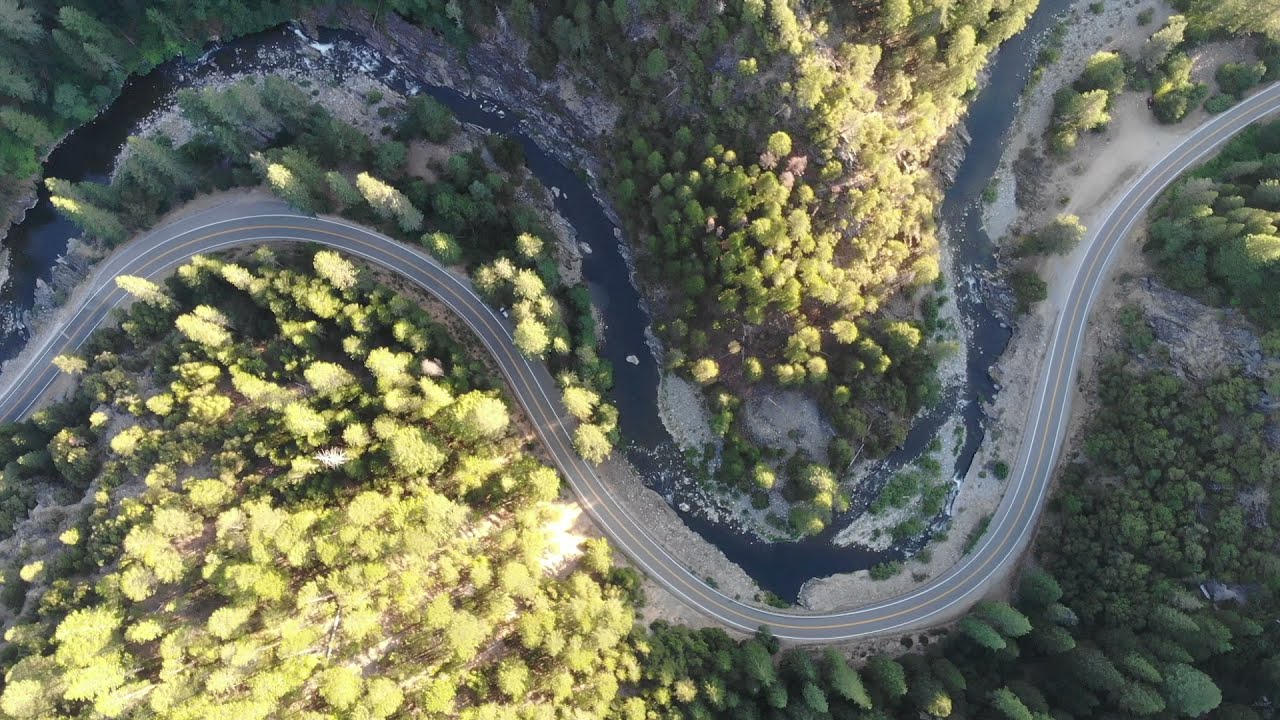This image captures a stunning aerial view of a winding, S-shaped, two-lane road snaking through a picturesque hilly region densely populated with lush, evergreen vegetation. Majestic cedar and pine trees, some reaching towering heights while others remain short, create a thick canopy that almost entirely obscures the ground below. Meandering alongside the road is a navy blue water body, possibly a river or stream, enhancing the natural beauty of the landscape. The road features several sharp curves, giving it a sinuous, snake-like appearance. Sunlight brightens the scene, casting a warm glow on the foliage, which is primarily composed of consistent green hues, although a patch of white vegetation—potentially flowering trees or shrubs—starkly contrasts against the greenery in the lower left-hand corner. This image, bathed in natural daylight, magnificently showcases the harmonious blend of rugged terrain and serene water features.